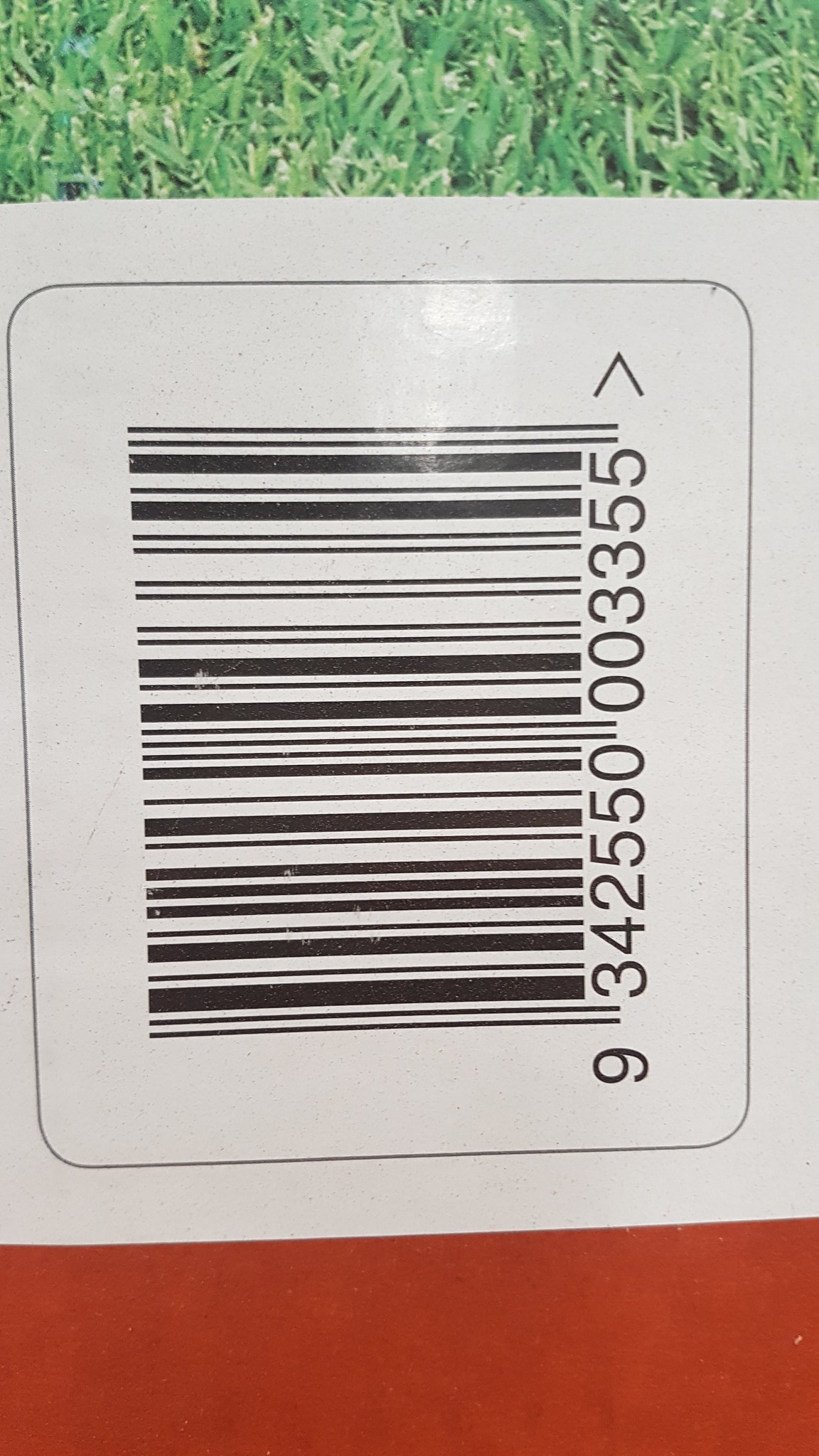The image depicts a product label featuring a prominent UPC barcode with the numbers 934-2550-003355, surrounded by a black border on a white background. Above the barcode, there is a printed picture of grass, suggesting it might be an outdoor or nature-themed item. Below the barcode, a vivid red stripe stretches horizontally across the label. An arrow is visible near the barcode, but it is pointing sideways due to the orientation of the photograph. The product label appears to have a glossy finish, reflecting light. Despite the detailed visual elements, the exact nature of the product remains unclear.